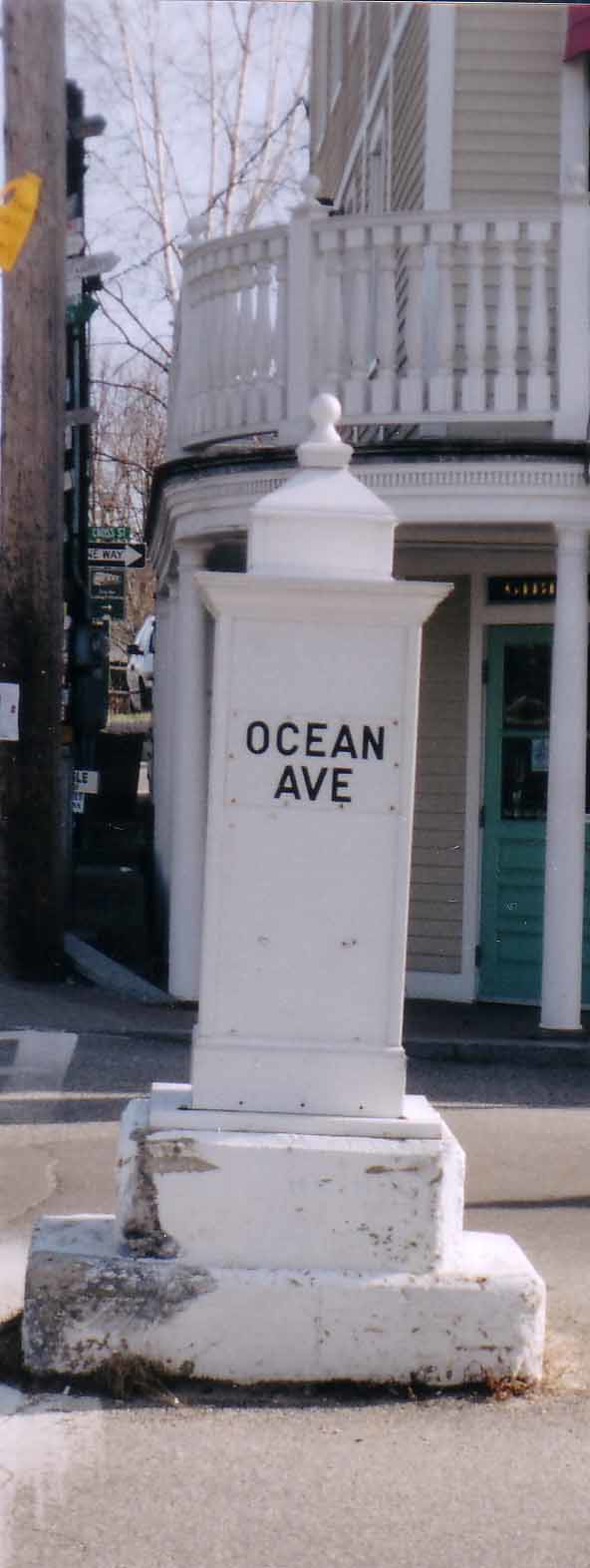The image showcases the picturesque corner of a charming two-story house, painted in a light beige hue and accented with pristine white trim. A generous wraparound porch adorns the upper level, providing an idyllic space for relaxation. Below, a vibrant green door stands out, inviting visitors into the cozy abode. The scene is set against a backdrop of a clear blue sky and a bare tree, signaling the presence of winter or early spring.

Adjacent to this charming house is a more utilitarian concrete building, offering a stark contrast. In the foreground, a street can be seen, adding an urban element to the setting. Dominating the streetside view is a substantial concrete sign, characterized by a large square base supporting another square section above it. This structure is crowned by a post featuring a decorative element that culminates in a small bowl. Emblazoned in bold black print on the sign is the designation "Ocean Avenue," marking the location with an elegant touch.